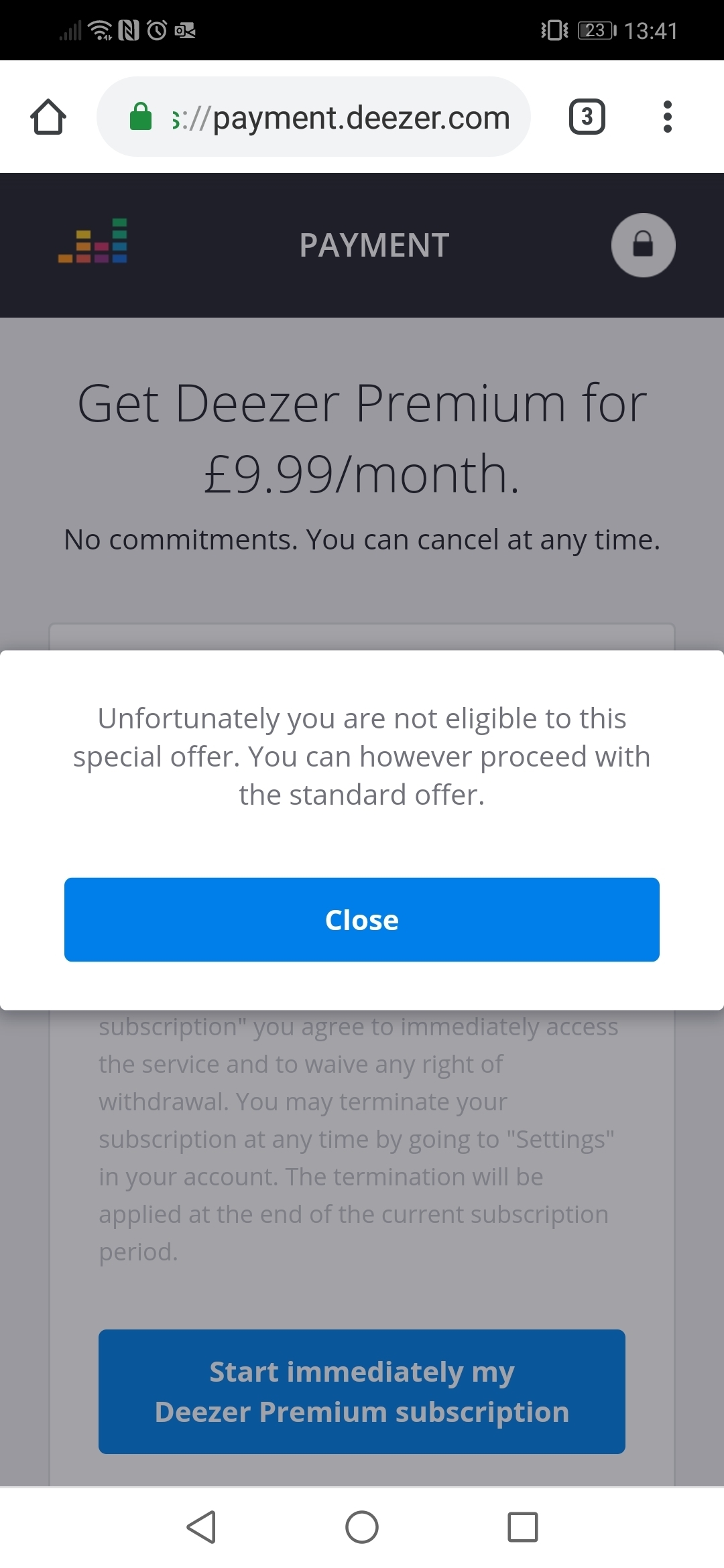This image displays a smartphone screen showing the website payment.deezer.com. At the very top, there is a tab indicator displaying the number '3', suggesting that three tabs are currently open. Next to this, a green lock icon signifies a secure connection. Below the URL, a pop-up message reads: "Unfortunately you are not eligible for this special offer. You can however proceed with the standard offer," accompanied by a blue close button.

The page advertises a subscription to Deezer Premium, stating: "Get Deezer Premium for £9.99 a month. No commitments. You can cancel at any time." Towards the bottom of the screen, there is a prominent button labeled, "Start immediately my Deezer Premium subscription." Additionally, navigation icons are visible including a back arrow, a centered black circle, and a black square at the bottom of the screen.

The website design features a white background with black text and a black navigation bar at the top. The Deezer logo, which resembles colorful sound bars in shades of orange, pink, purple, green, and blue, is prominently displayed at the top of the page. The top of the smartphone screen also shows standard indicators such as the time, battery percentage, and a clock icon, typical elements of a mobile web interface.